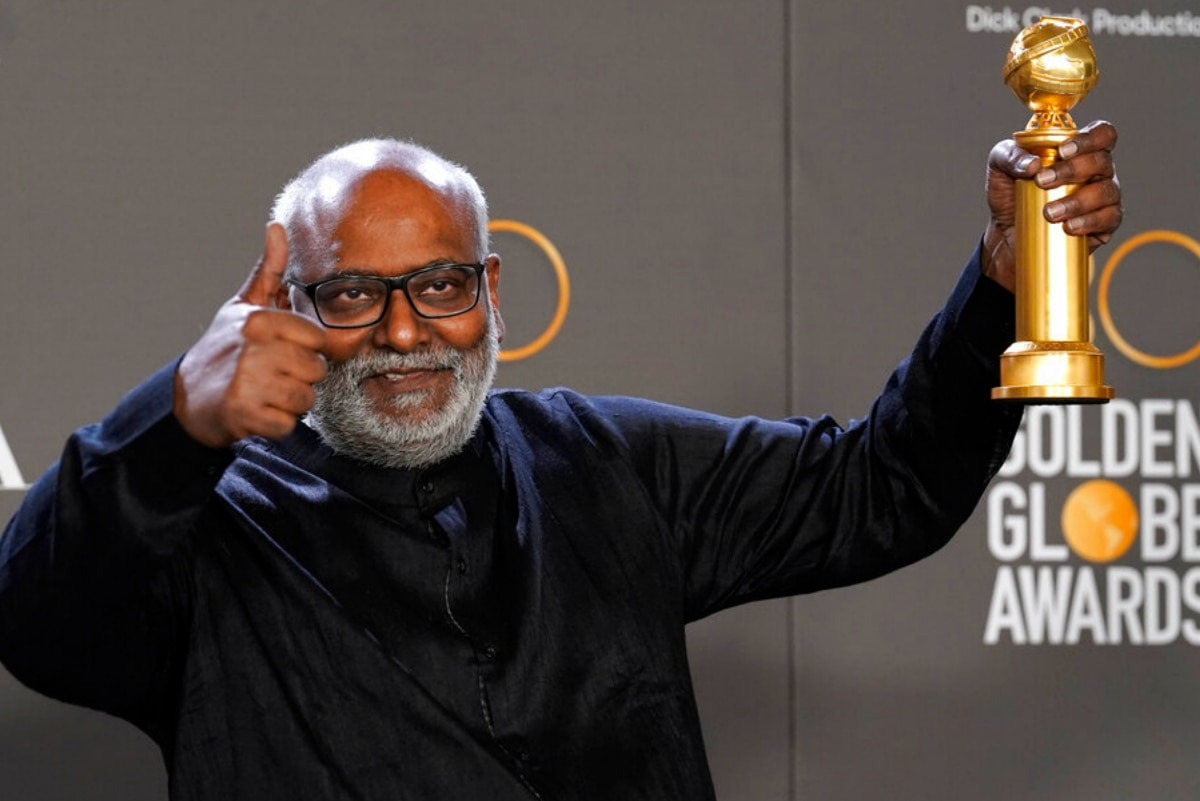In this celebratory photo from the Global Golden Globe Awards, an older Black man, who appears to be a director, is proudly holding up his Golden Globe trophy in his left hand while giving a thumbs-up with his right hand. He stands in front of a step and repeat banner adorned with the Golden Globe Awards logo and the faint branding of Dick Clark Productions. The award's long, gold-colored base is topped with a golden sphere. The man has a bald head with white hair on the fringes, a full white beard, and a mustache. His brown eyes are framed by black-rimmed glasses, and he is wearing a dark-colored, possibly black, zip-up long sleeve jacket. His joyful expression is mirrored by his body language, capturing a moment of triumph and happiness.